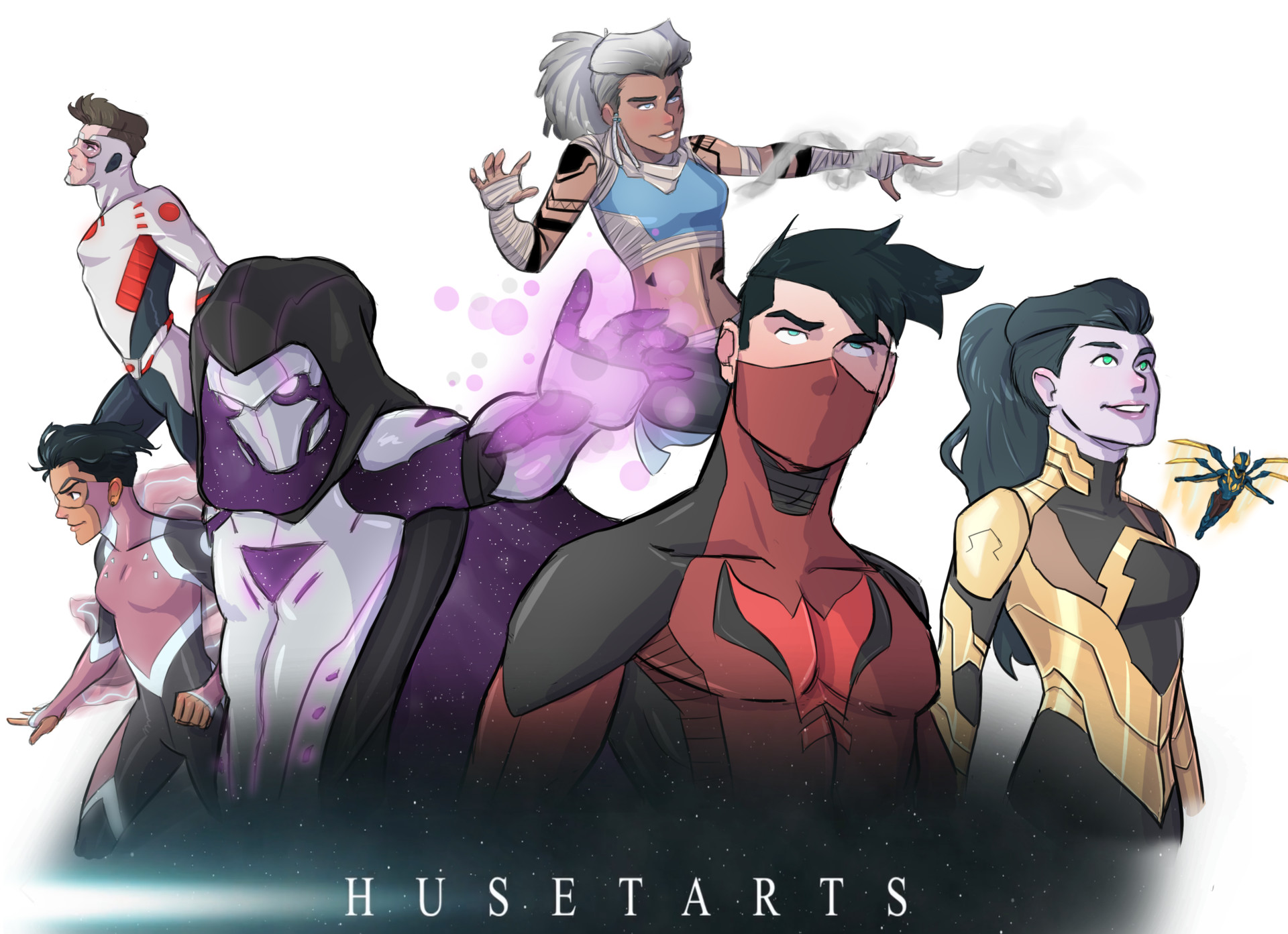This comic book-style illustration titled "HUSETARTS" showcases seven distinct superhero figures. The title is prominently displayed in bold white text at the bottom of the image, set against a starry backdrop. 

From left to right: 

1. **Red and White Male Hero**: A male superhero dressed in a white and red outfit. He has brown hair, goggles, and a costume with black accents on his back.
   
2. **Pink and Gray Female Hero**: Next is a female hero with a light brown or black hair styled short. She wears a pink, white, and dark gray costume.
   
3. **Cloaked Villain**: Following her is a mysterious figure in a dark hooded cloak with a metallic mask that has glowing purple eyes and a purple triangle on the chest. This character has a ghostly, transparent purple arm stretched out menacingly.
   
4. **Red-costumed Male Hero**: Then there is a white male hero with striking blue eyes and black hair, wearing a red suit similar to a famous movie character, with black accents on his shoulders and a bat-like emblem on his chest.
   
5. **Brown and Tan Armored Female Hero**: Beside him stands a young woman with black hair in a ponytail, blue eyes, and a costume reminiscent of armor in shades of tan, dark brown, and light brown.
   
6. **Silvery-haired Smoke Manipulator**: Centered at the top is a female hero with silvery hair and brown skin. She is wrapped in what looks like white bandages and has a cloud-like snake encircling her arm, as smoky tendrils waft from her hands.

7. **Tiny Flying Fairy-like Superhero**: Off to the side, a tiny superhero that resembles a fairy with dragonfly-like wings floats. This character has a blue and yellow costume, further emphasizing a bug-like appearance.

Each character showcases unique and vivid design elements, contributing to the compelling composition of the "HUSETARTS" tableau.